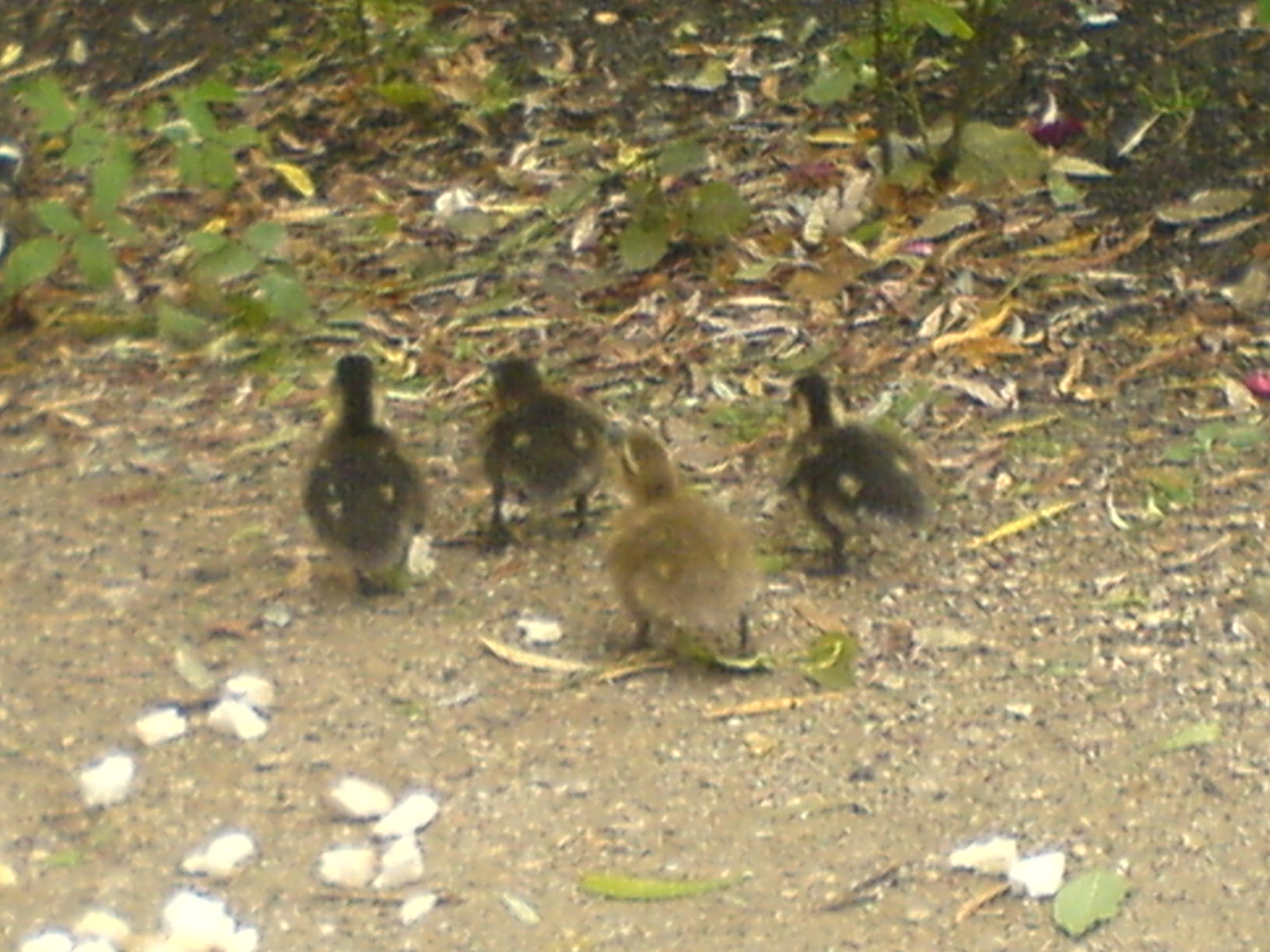The image captures a group of four ducklings walking away from the camera on a dirt and pebble-strewn path. The scene is bright and well-lit, though slightly out of focus. The ducklings' soft feathers suggest they are young. In the foreground, two dark brown ducklings with webbed feet lead the group. Behind them, another duckling with light, fluffy, brown feathers follows. The fourth duckling, on the far right, is similar in appearance to the two in the front but features a lighter brown on its back and a small white underside. The ground they tread is scattered with pebbles, rocks, and white chunks that could be broken leaves or stones.

Surrounding the dirt path are various fallen leaves in shades of yellow, brown, and green, with a few remaining on their plants on the upper left-hand side of the image. The background holds more leaf-covered ground with hints of green weeds and wildflowers. The overall ambiance is natural, giving a sense of the ducklings’ journey into a woodsy area.